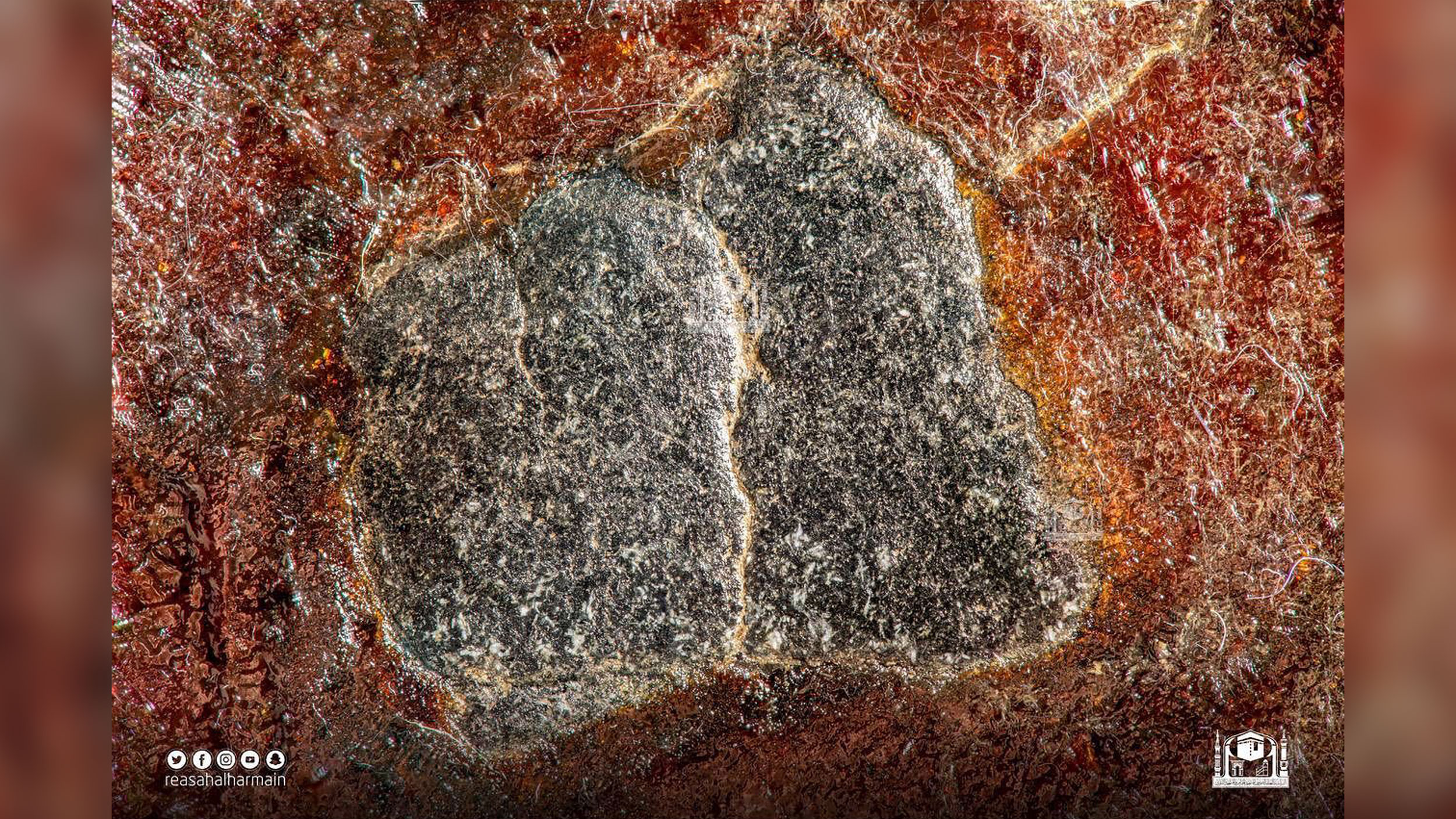The photograph captures a remarkably detailed image of what appears to be two gray and black rocks with various intersecting white cracks. These rocks are nestled within a surrounding matrix of semi-transparent, red, amber-like material, giving the entire scene a rugged and natural appearance. The surface of the assemblage is notably rough, with the white lines and cracks extending over both the rocks and the amber encasement. The composition is accentuated with additional colors, including subtle hints of blue. At the bottom left corner, a watermark featuring white text and various social media logos reads "Ria Sahal Harmein." On the bottom right corner is a crest depicting a white palace, serving as another distinctive logo. This intricate arrangement of rocks and amber, combined with the detailed text and logos, makes for a visually compelling and richly textural image.